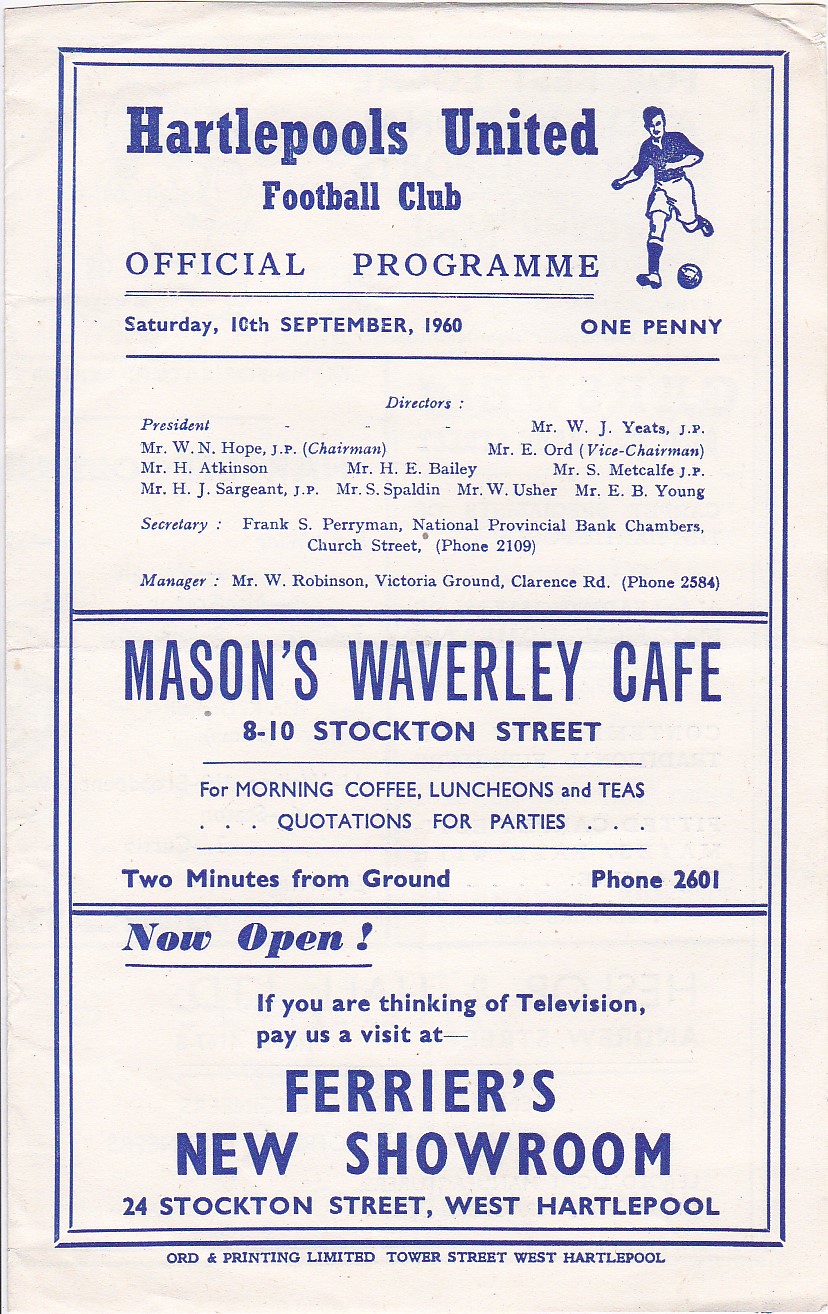This image showcases an antique, pink-hued pamphlet, most likely dating back to September 10, 1960. The pamphlet, adorned in blue text, is an official program for the Hartlepool's United Football Club. The header prominently displays the club's name and the words "Official Program," followed by the date and the price, one penny. To the right of this text is an illustration of a professional athlete kicking a soccer ball. 

Below the title, there is a detailed list of the football club's directors, including the president, secretary, and manager. 

Further down, the pamphlet features an advertisement for Mason's Waverly Cafe, located at 810 Stockton Street. The ad touts offerings such as morning coffee, luncheons, and teas, with a special note mentioning quotations for parties and that the cafe is just two minutes from the football ground. Contact details provided include the phone number 2601.

At the bottom of the page, another advertisement invites readers to visit Farrier's New Showroom at 24 Stockton Street, West Hartlepool, if they are considering purchasing a television. The advertisement claims that the showroom is "now open."